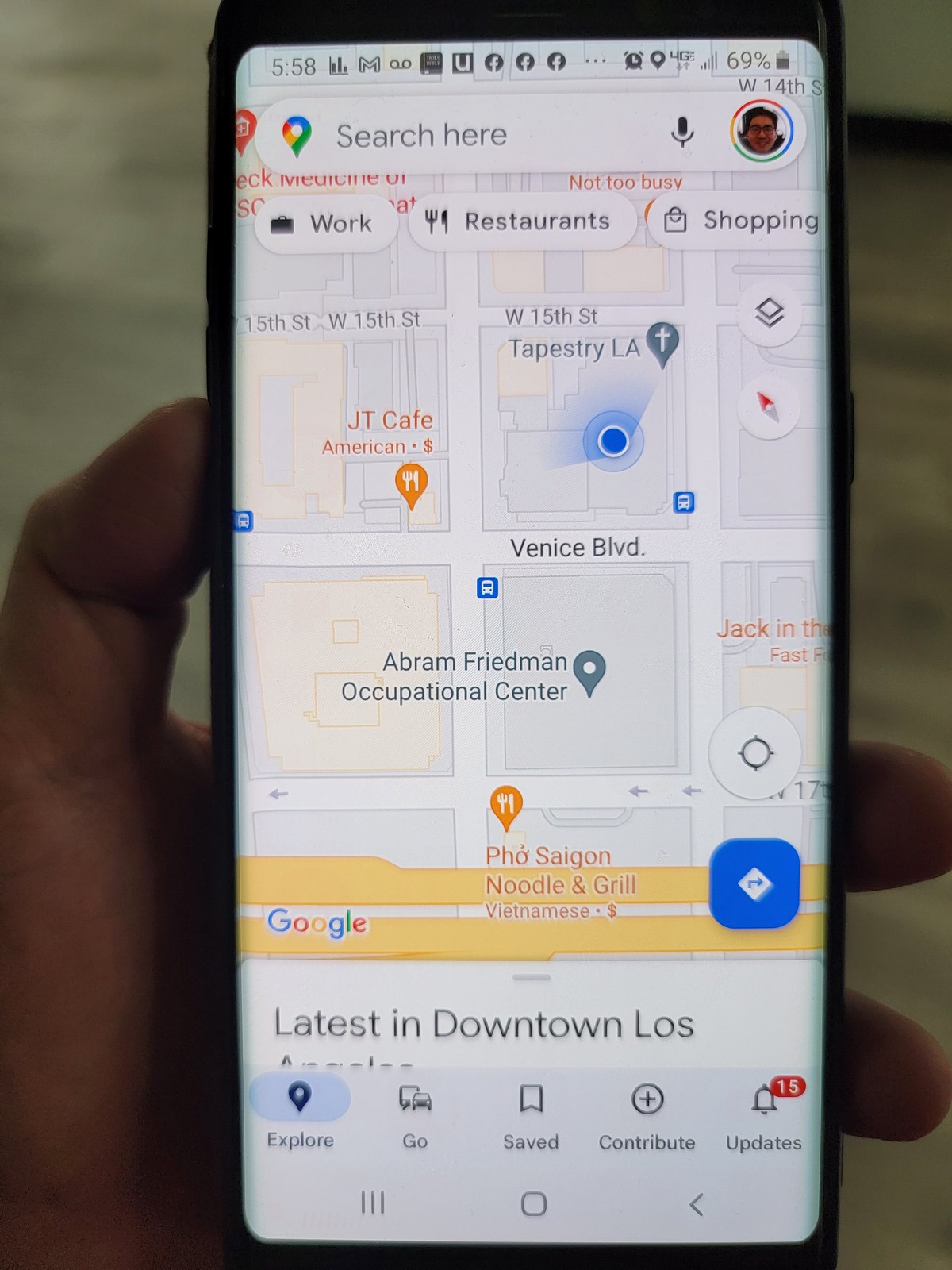A detailed photograph captures a person holding a smartphone in their left hand, prominently displaying the device's screen. On the screen, a map is visible, showcasing various locations and establishments. The top menu bar indicates the time as 5:58 and displays icons for Facebook, an alarm clock, and a battery status of 69%. Below this, a search bar featuring the Google logo and a microphone icon is present, alongside a small profile photo of a man on the right side.

The map highlights a number of locations: JT Cafe (categorized as American cuisine), Venice Boulevard, Tapestry LA, 15th Street, West 15th Street, Abraham Friedman Occupational Center, Pho Saigon Noodle and Grill (Vietnamese cuisine), and Jack in the Box (fast food). At the bottom of the map, a partially visible text reads, "Latest in downtown Los..." but is cut off.

The bottom menu bar of the screen includes five options: Explore, Go, Saved, Contribute, and Updates, with the Updates section showing 15 notifications. The background of the image is softly out-of-focus and appears to be beige-colored carpeting.